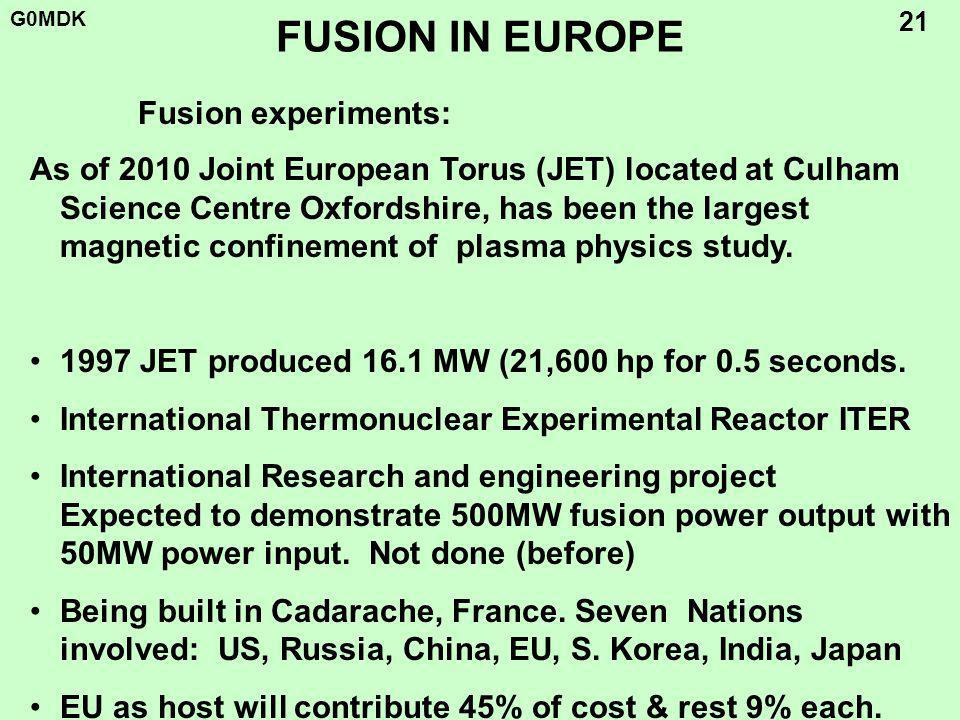The image is a green rectangular slide with a light green background featuring all black text. In the upper left corner, it prominently displays "G0MDK," and the upper right corner has a "21." The center top title reads "Fusion in Europe." Below the title, in smaller font, it states "Fusion Experiments as of 2010." The text details that the Joint European Taurus (JET), located at Culham Science Center, Oxfordshire, is the largest magnetic confinement plasma physics study. A series of bullet points follow:

- In 1997, JET produced 16.1 MW (21,600 HP) for 0.5 seconds.
- The International Thermonuclear Experimental Reactor (ITER) is an international research and engineering project expected to demonstrate 500 MW fusion power output with a 50 MW power input, a feat not previously accomplished.
- ITER is being built in Cadarache, France, involving seven collaborating nations: the US, Russia, China, the EU, South Korea, India, and Japan. The EU, as the host, will contribute 45% of the cost, while the other countries will contribute 9% each.

This slide provides a concise and detailed overview of significant milestones and collaborative efforts in European fusion experiments.